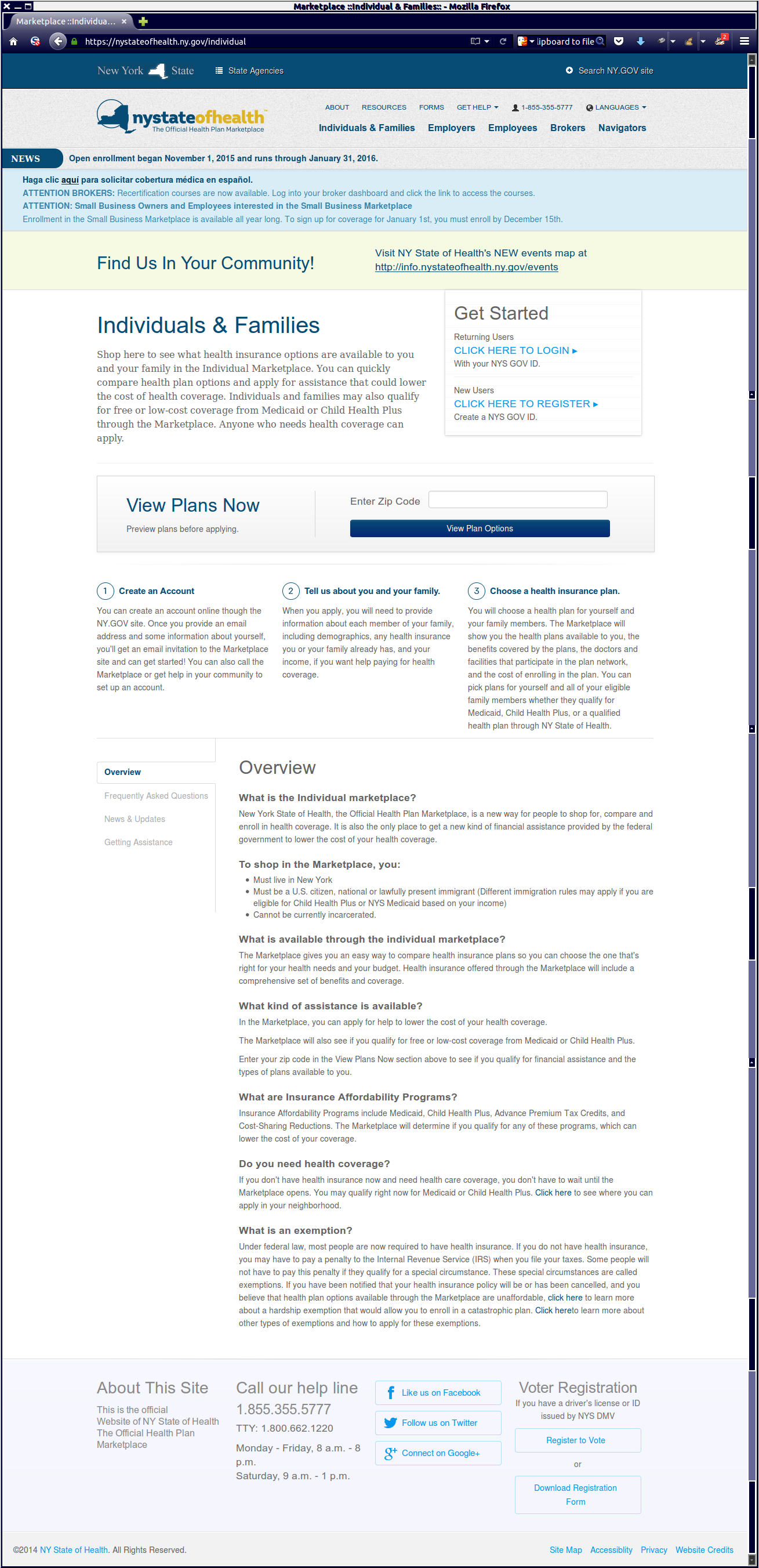In this image, we see a snapshot of a website displayed in a browser, indicating a single tab open. The website belongs to the New York State and prominently features the New York State of Health logo and title in the top left corner. Adjacent to the logo are several navigation categories in blue text: Individuals and Families, Employers, Employees, Brokers, and Navigators.

Below the navigation bar, a light blue background highlights important announcements: "Attention Brokers," "Attention Small Business Owners and Employees," and "Interested in the Small Business Marketplace?" This section also directs users to "Find Us in Your Community" with a link to New York State of Health News Events Map at http://info.newyorkstateofhealth.ny.gov events.

Further below, there is another section titled "Individuals and Families." To the right, a small box offers links for new and returning users: "Get Started" for new users and "Click Here to Log In" (in blue text) for returning users.

Centrally located on the page, three numbered steps guide users through the process of obtaining health insurance:
1. Create an Account
2. Tell Us About You and Your Family
3. Choose a Health Insurance Plan

Further down the page, the word "Overview" appears, indicating the beginning of additional explanatory content.